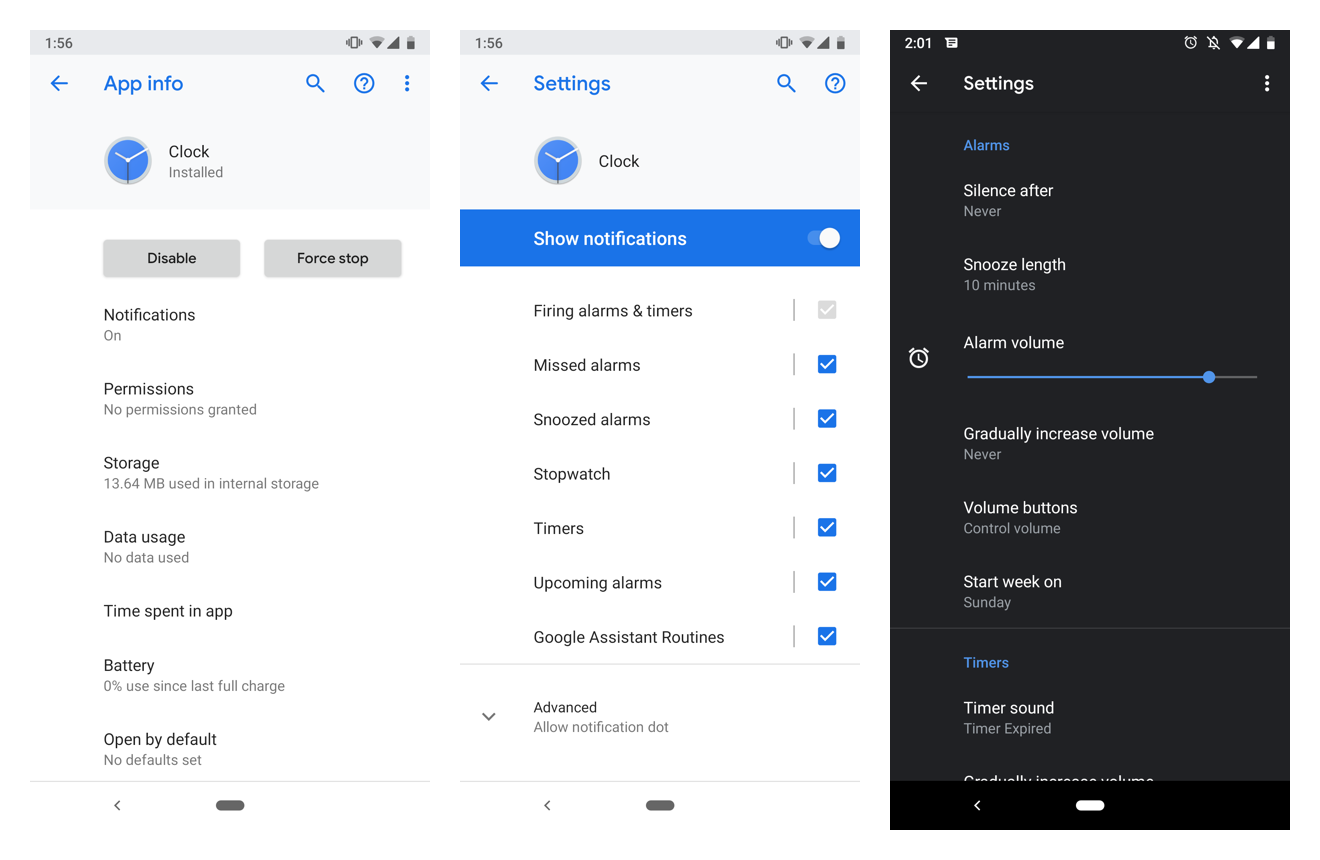This is a sequence of three horizontally arranged smartphone screenshots detailing various settings for a clock app. 

The first screenshot provides an overview of the "App Info" for the Clock app, identified by its blue icon featuring white hour and minute hands, and a black second hand. The app details include options such as "Disable" and "Force Stop," with notifications turned on. It lists no permissions granted, and specifies storage usage as 13.64 MB in internal storage. The data section indicates no data used and specifies the time spent in the app. The battery section shows 0% usage since the last full charge. Additionally, there is a note that the app is not set to open by default.

The second screenshot displays the detailed "Settings" for the Clock app. The shortcuts and settings under this category show that notifications are enabled, delineated by the slider being turned on. Different notification categories are checked, including "Firing alarms and timers," "Missed alarms," "Snoozed alarms," "Stopwatch," "Timers," and "Upcoming alarms," indicating they all will trigger alerts. The last option checked is "Google Assistant routines." The "Advanced" section mentions the "Allow notification dot" feature.

The final screenshot continues under "Settings," specifically focusing on "Alarms." Detailed configurations include "Silence after" which is set to "never," a snooze length of 10 minutes, and an alarm volume slider positioned near maximum volume. The "Gradually increase volume" feature is turned off while the "Volume buttons" setting is configured to control the volume. Additional settings include starting the week on "Sunday," and various timer settings including "Timer sound" and "Timer expired," with a partially visible option "Gradually increase volume," suggesting more settings at the bottom that are cut off in the image.